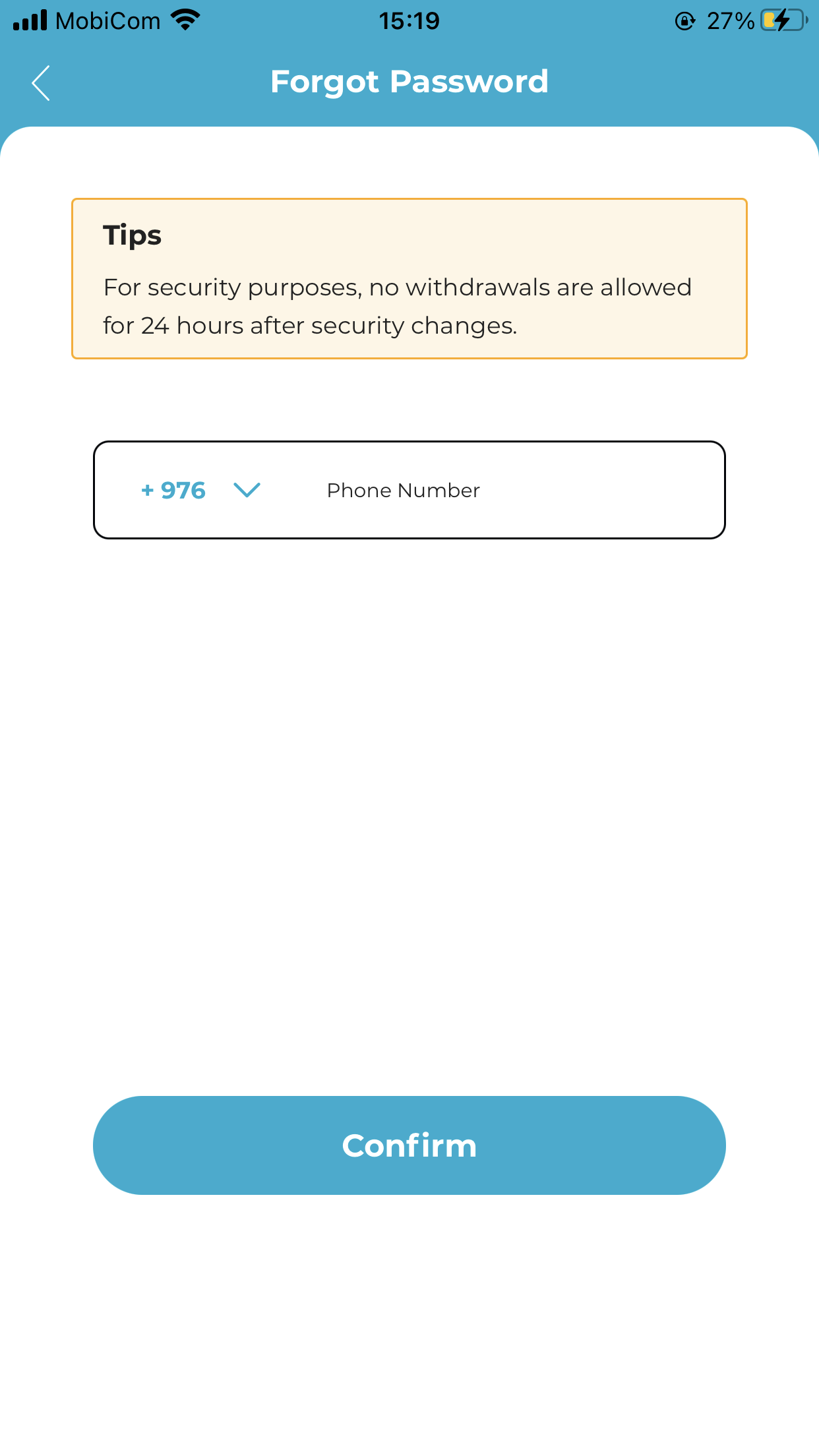The screenshot features a mobile application interface with a layout consisting of a light blue header and a white body with rounded top corners that slightly overlap the blue header. At the top of the header, there are several black icons: to the left, five vertical black bars of increasing height indicating signal strength; in the center, the bold black text "MobiCom"; and to the right, a black Wi-Fi icon. Below these icons, a thin white arrow pointing left is located on the left side, and centrally positioned white text reads "Forgot Password."

The body of the page displays a pale yellow rectangle with a thin orange outline at the top center. Inside this rectangle, the word "Tips" is written in bold black text in the top left corner, followed by two lines of thin black text: "For security purposes, no withdrawals are allowed for 24 hours after security changes."

Below this, there is a white rectangle with rounded corners and a thin black outline. On the left side of this rectangle, there is a blue "+976" followed by a downward-pointing arrow. The center of the rectangle contains small black text reading "Phone Number."

A large area of negative white space separates the phone number field from a teal, pill-shaped button at the bottom of the page. This button features white text in the center that reads "Confirm." Finally, there is a slight amount of white space remaining beneath the button to the bottom of the page.